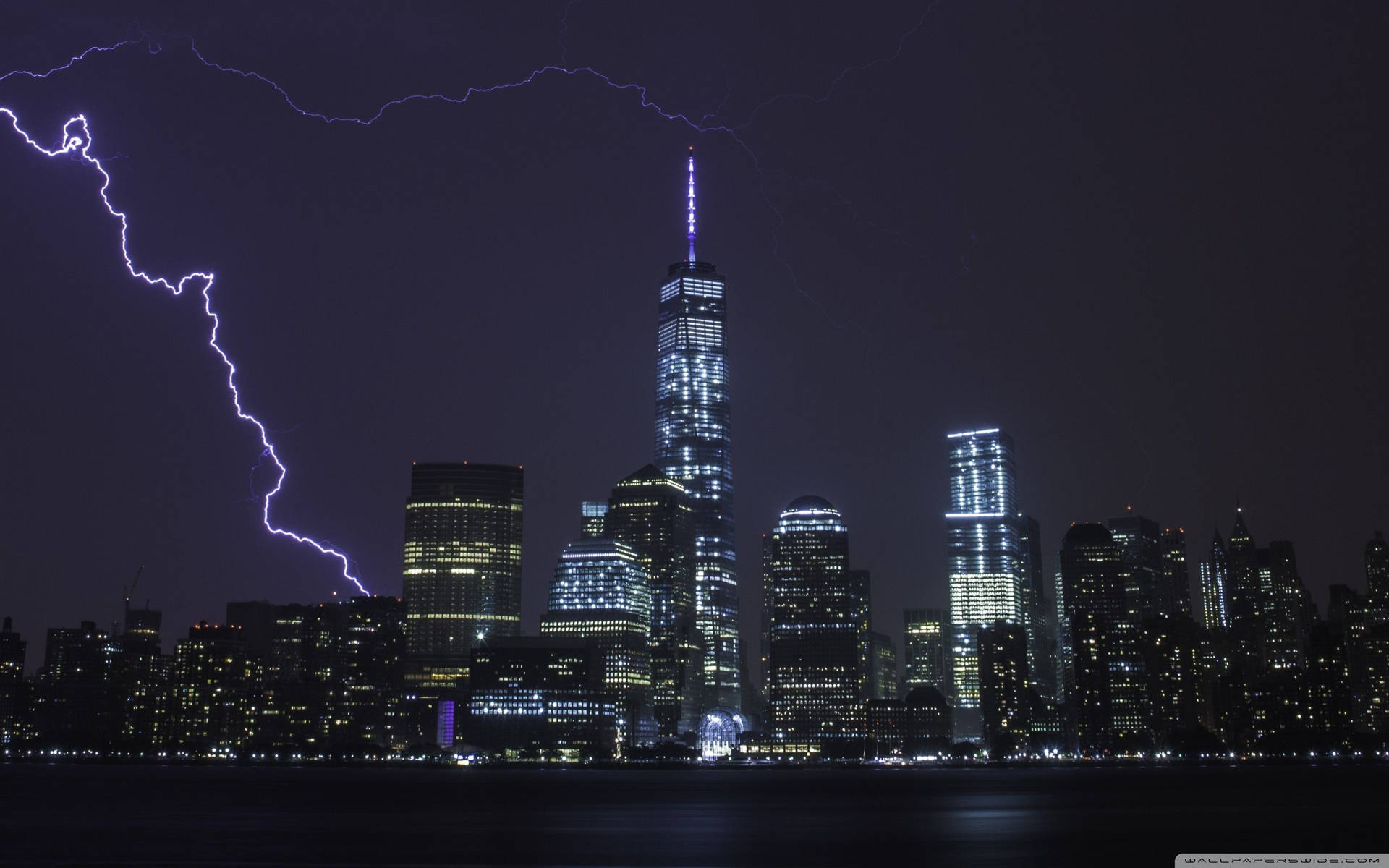This is a striking nighttime photograph of the Manhattan skyline, likely taken from New Jersey, showcasing a dramatic dry electrical storm. The image primarily features a skyline dominated by a very tall skyscraper centrally located, equipped with a brightly lit needle or radio tower. Surrounding this imposing structure are smaller skyscrapers, illuminated in shades of yellow, blue, and various other colors. The sky, a mix of dark and purplish hues, is starkly contrasted by two distinct arcs of lightning. One strong, bright bolt strikes towards the city on the left side of the photograph, while a thinner, fainter lightning streak arcs above the skyline and stretches toward the middle of the sky before fading out. The photograph appears to be a long exposure shot, as evidenced by the smooth surface of the Hudson River in the foreground. The overall blue and purple tones suggest post-processing enhancements to amplify the dramatic and somewhat eerie atmosphere of the scene, resulting in a very professional and visually compelling image.